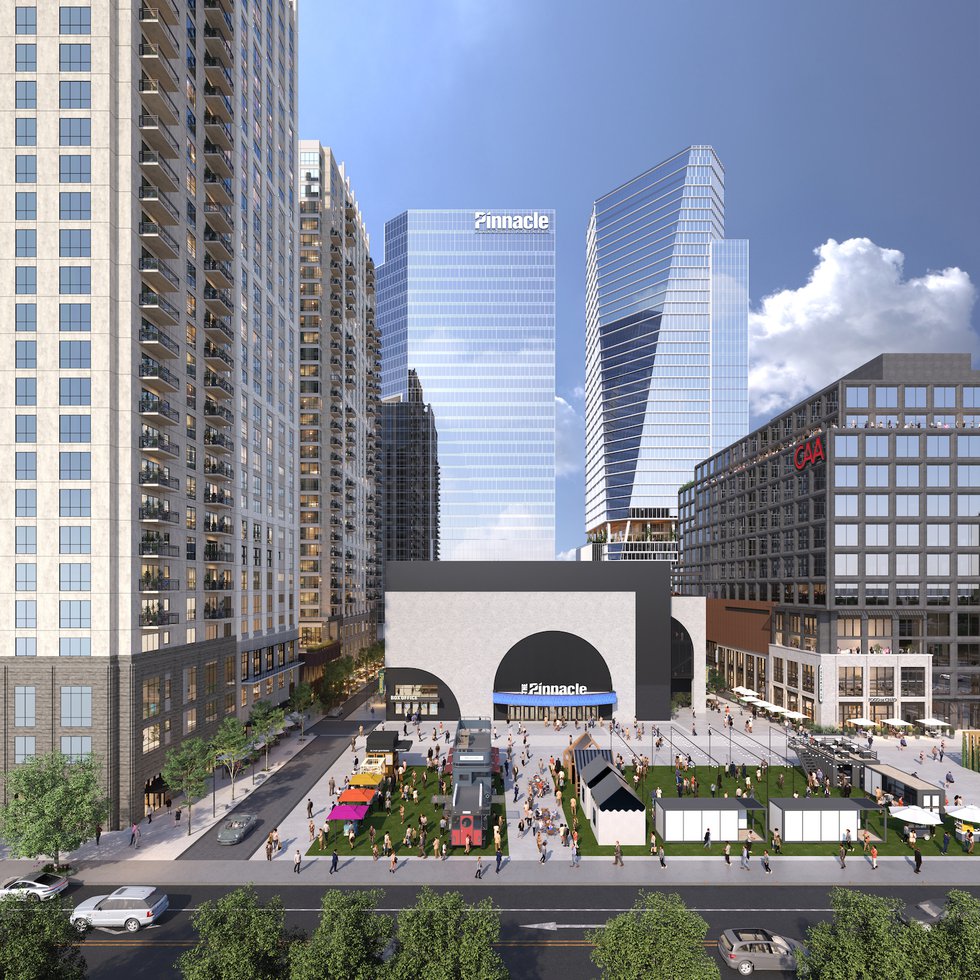The image is a 3D color-rendered architectural elevation of an urban scene in portrait orientation, depicting the new music venue, The Pinnacle, in Nashville, Tennessee. Central to the image is a tall, square skyscraper with mirrored walls emblazoned with the white sign reading "Pinnacle" in the top right corner. Adjacent to it on the right is another skyscraper of a similar design but slightly taller and distinctive for its fan-shaped facet. The left side features two beige high-rise buildings with a stucco finish, adorned with multiple balconies on each level.

In the foreground, there is a bustling city street with asphalt and marked lanes, containing several cars and populated with green-leafed trees. The ground level reveals a gray and white building also named Pinnacle, indicated by white signage and a blue canopy. Smaller structures with shops and pop-up tents populate a large courtyard below, where numerous people are seen walking and browsing, creating a dynamic, lively atmosphere. Additionally, a shorter building with "CAA" in red lettering on its top right is visible on the right side of the image.

The overall scene provides a detailed and vibrant depiction of the urban environment, emphasizing the towering, glass-paneled buildings and active street life below.